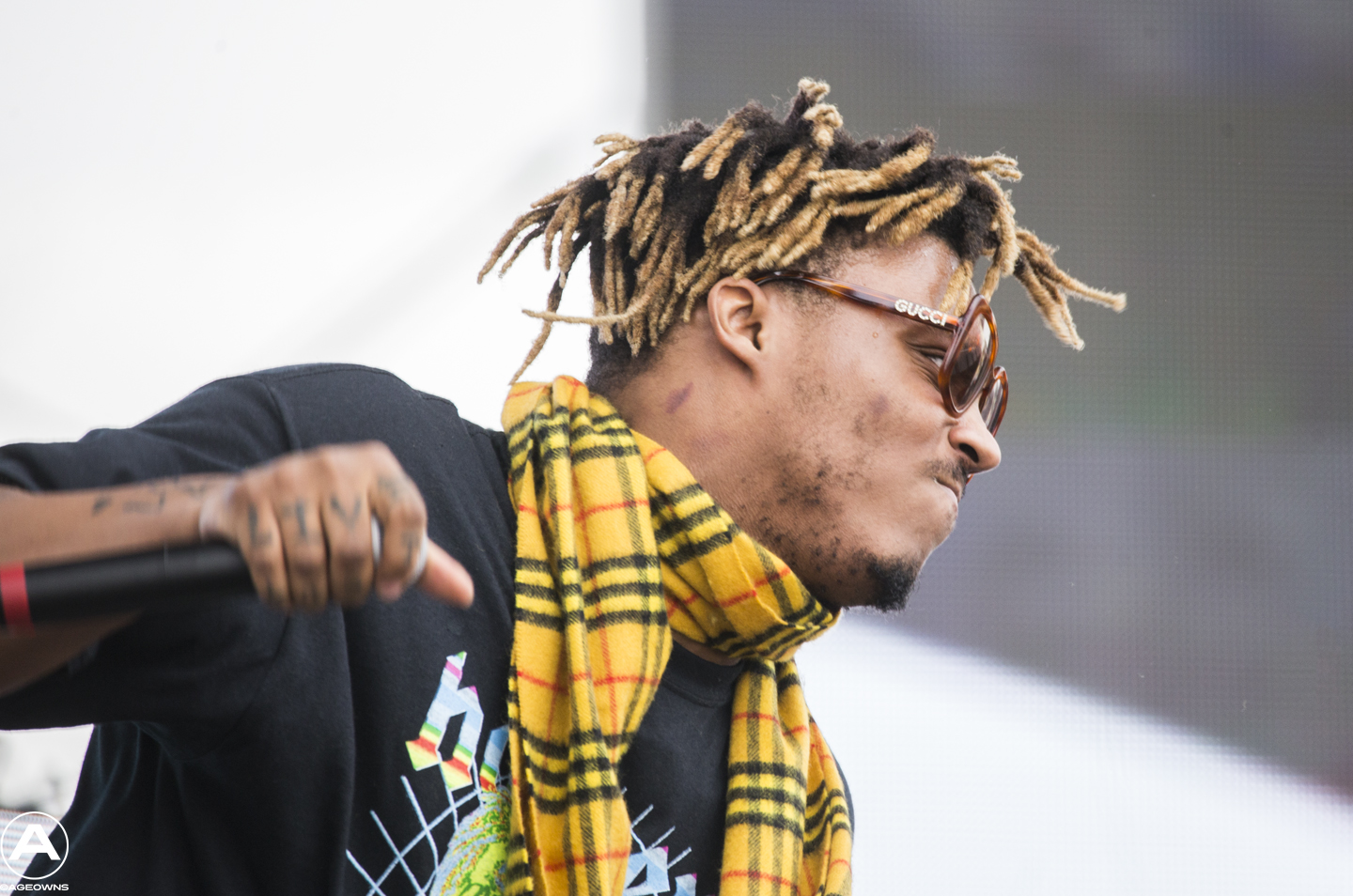The image depicts a young light-skinned black man with short, dark hair that transitions into light blonde tips styled in dreadlocks. He appears to be performing at an outdoor concert in the middle of the day, evidenced by his intense expression and dynamic posture, which suggests he is mid-performance. He holds a microphone in his right hand and seems to be making a punching motion, adding to the energy of the scene. A vivid yellow scarf with black and red stripes adorns his neck, contrasting with his short-sleeved blue t-shirt, which features a rainbow mirror-effect logo or text across the chest. His stylish look is completed with Gucci sunglasses and visible tattoos on his knuckles and forearms. The blurred outdoor background contains shades of gray and white, indicating a lack of specific details but reaffirming the open-air setting.